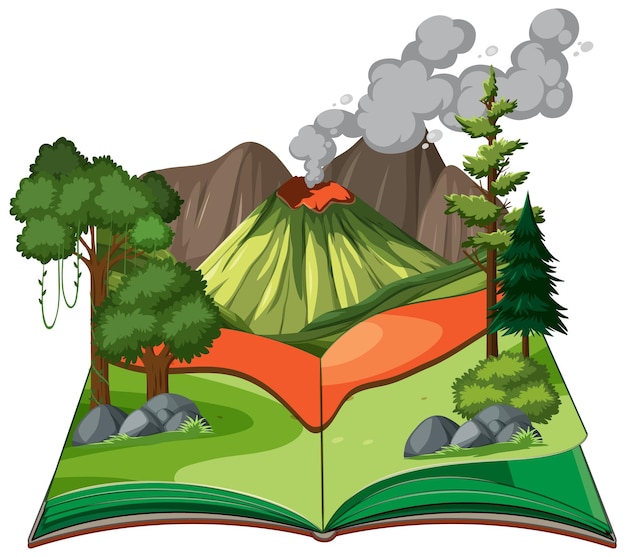This cartoonish illustration depicts a children's pop-up book opened to the middle with vibrant green pages. The central feature is a green volcano, with orange lava flowing down its sides, highlighted by an orange banner draped into the spine of the book. Gray smoke billows from the volcano’s peak, enhancing the sense of eruption. Behind the volcano, a range of brown mountains or hills spans the background. In front of the volcano, varied greenery is displayed: on the left page, two trees with brown trunks and rocks at their bases stand tall, and on the right page, there's a pine tree, an evergreen, and a shrub, all also accompanied by rocks. The scene is richly textured with a combination of different shades of green and the vivid depiction of natural elements, making it a captivating and detailed portrayal typical of children's literature.